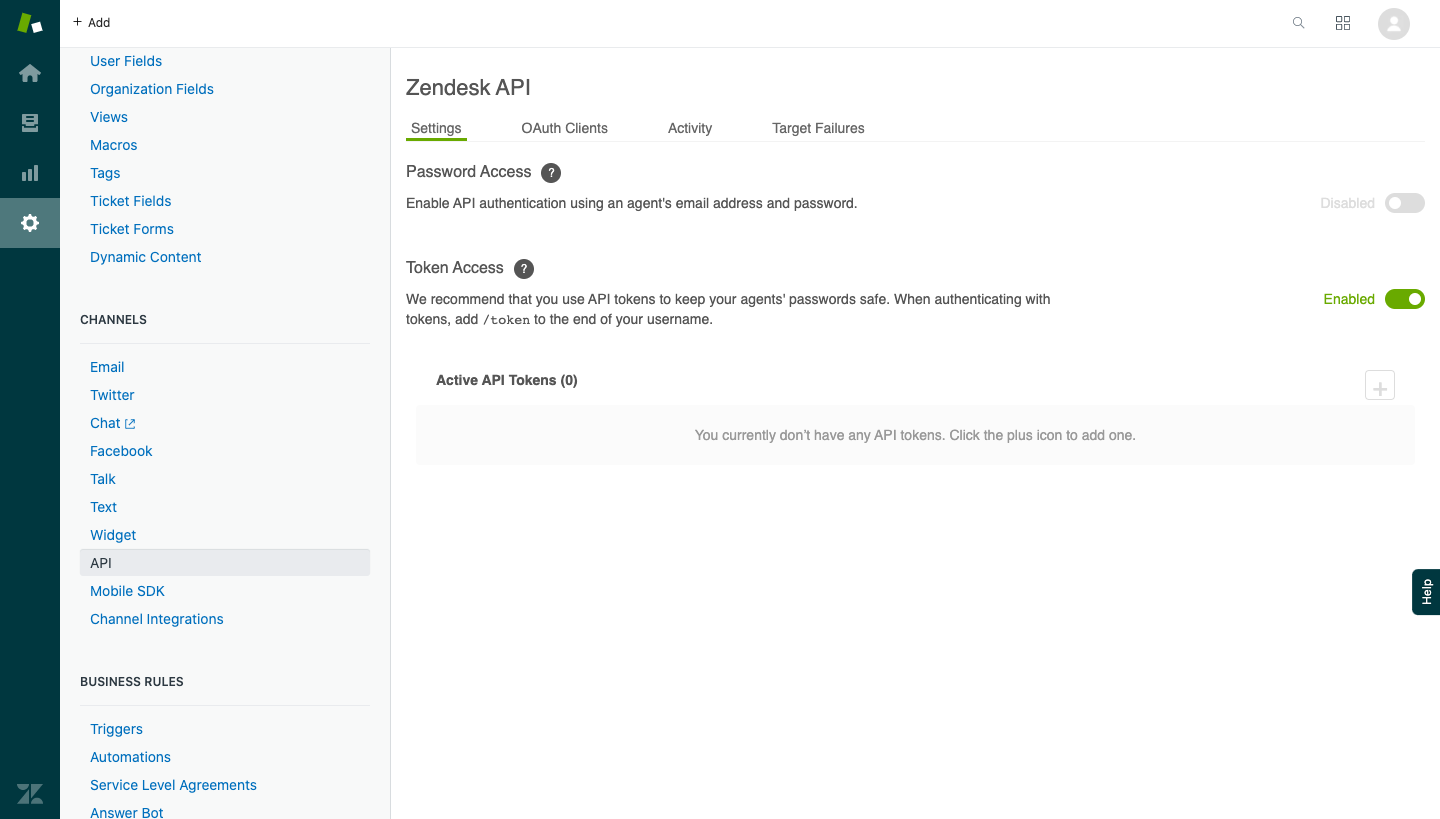Screenshot of the **Zendesk Desk API Settings Page**:

On the left-hand side of the screen, there's a vertical blue navigation banner. This banner includes icons arranged vertically: a home icon, a gear icon representing settings (which is selected), three horizontal lines, and a folder icon. 

Under the selected settings icon, a list of available options is displayed: 
- User Fields
- Organization Fields
- Views
- Macros
- Tags
- Ticket Fields
- Ticket Forms
- Dynamic Content

Below these options is a header labeled **Channels**, under which the following channels are listed:
- Email
- Twitter
- Chat
- Facebook
- Talk
- Text
- Widget
- API
- Mobile SDK
- Channel Integrations

Further down, another header titled **Business Rules** appears with the following options:
- Triggers
- Automations
- Service Level Agreements
- Answer Bot

The **API** section is currently selected.

In the main content area of the screen, the top header reads **Zendesk API** with four tabs below it:
- Settings
- OAuth Clients
- Activity
- Target Failures

The **Settings** tab is selected. The content under this tab includes:

1. **Password Access**: 
   - Labeled with a question mark in a circle for additional information.
   - A description reads: "Enable API authentication using an agent's email address and password." 
   - A switch to enable or disable this feature is present on the right, and it is currently disabled.

2. **Token Access**: 
   - Also labeled with a question mark in a circle for additional information.
   - It states: "We recommend that you use API tokens to keep your agent's password safe when authenticating with tokens. Add /tokens to the end of your username."
   - A switch to enable or disable this feature is on the right and is currently enabled, indicated by green text reading "Enabled."

3. **Active API Tokens**:
   - It notes: "You currently do not have any active API tokens. Click the plus icon to add one."
   - A plus icon is present to the right, ready to be used for adding new API tokens.

This detailed view of the Zendesk Desk API settings page provides a comprehensive overview of the available options and current configuration.